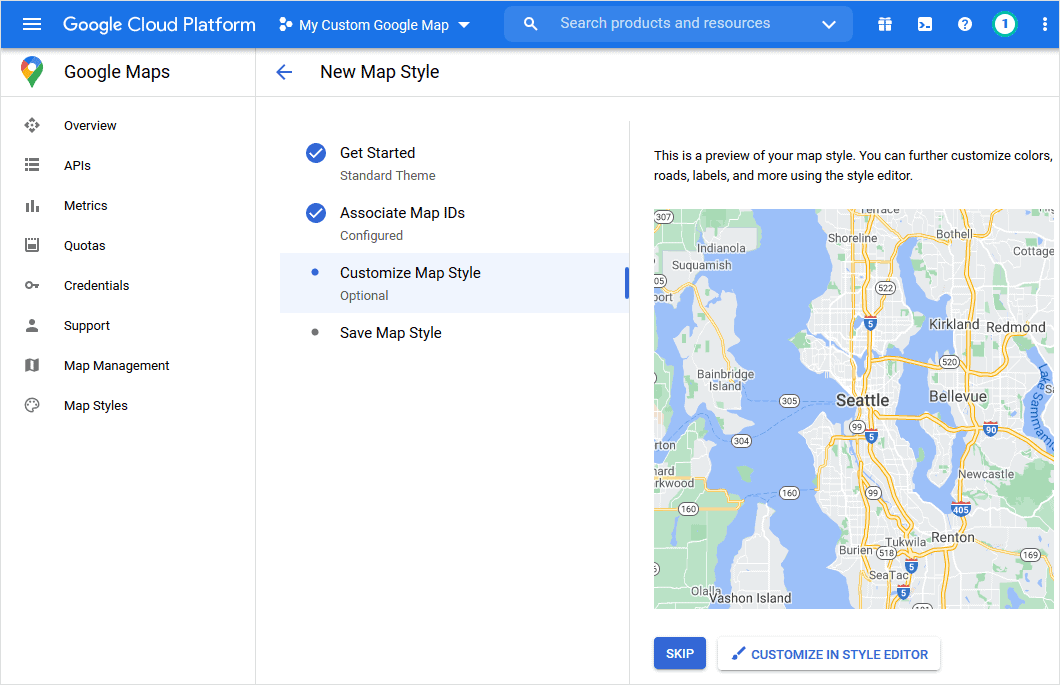**Detailed Descriptive Caption:**

The image depicts a user interface from Google Cloud Platform, specifically focused on creating a custom Google Map. The primary interface shows the title "My Custom Google Map," with an empty search bar below it. On the left-hand side, a menu lists various options aligning vertically: "Google Maps, Overview, APIs, Metrics, Quotas, Credentials, Support, Map Management, and Map Styles."

At the top of the interface, directly beneath the Google Maps logo, there is a blue arrow indicating the option "New Map Style." Below this, there are two items marked with blue check circles: one labeled "Get Started" and the other "Associate Map IDs," both marked with check marks, indicating their completion. Under the "Configured" section, another task is similarly checked off.

The process appears to involve customizing the map’s style, though this step has not been completed yet. On the third section, a preview of the map style is displayed. This preview highlights an area around Seattle, showcasing standard map elements such as highways and bridges. A note in this section informs the user that they can further customize specific features like colors, roads, and labels using the Style Editor.

The map currently looks like a standard representation with the highlighted areas and infrastructure, anticipating further customization.